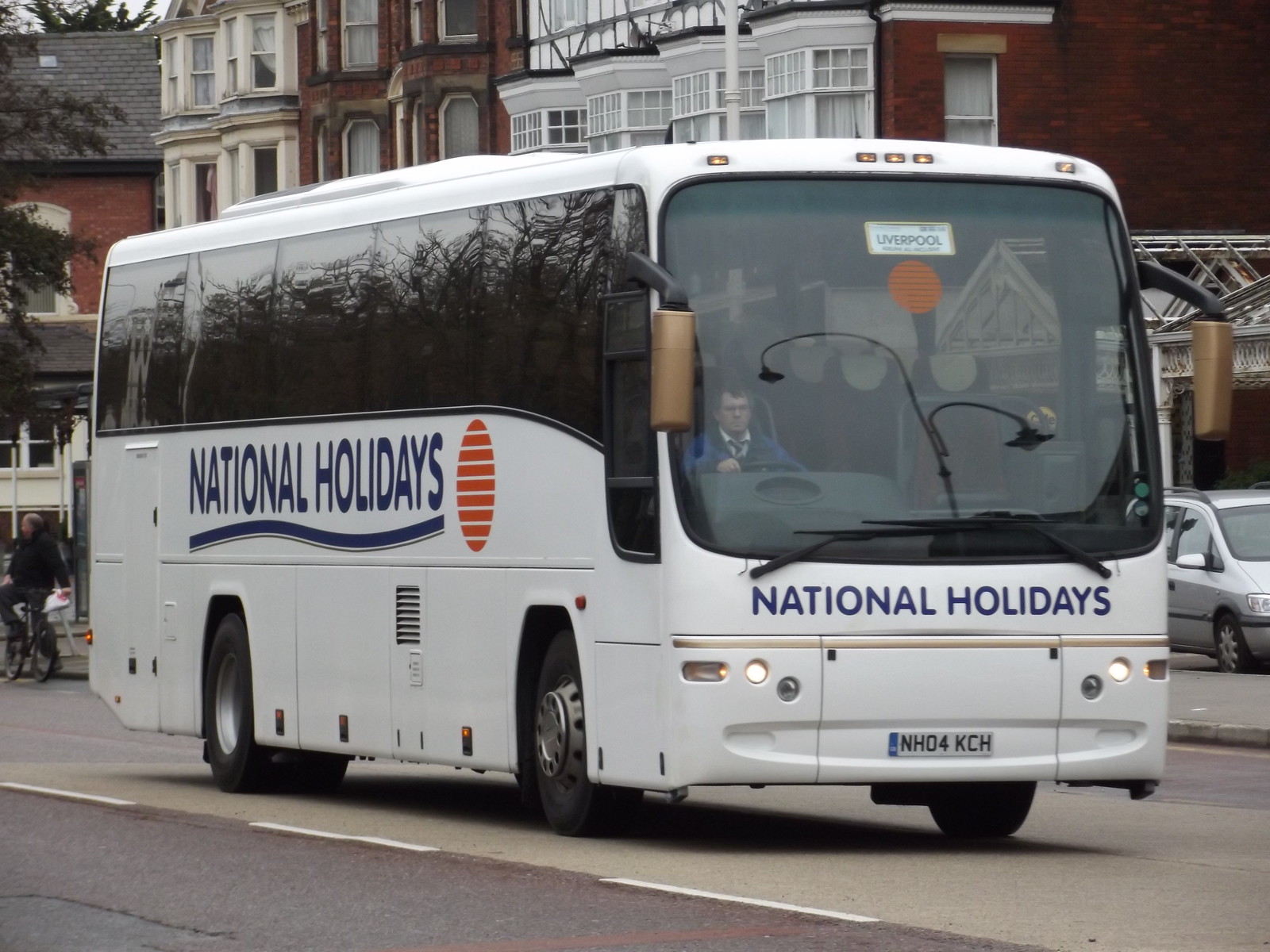The image is a color photograph taken outdoors on a busy city street. Dominating the scene is a large white bus with prominent smoked glass windows. The bus has "National Holidays" written in large navy blue letters on its side and front, underlined by a blue wave. An orange sun-like circle logo accompanies the text. The front placard reads "Liverpool," indicating its destination. The driver, seen through the bus's expansive front windshield, is wearing a blue jacket, white shirt, and possibly a tie. The bus's license plate reads NH04 KCH.

The bus is positioned moving from right to left across the image, prominently featuring its front and right sides. The street comprises several lanes with a dotted white dividing line. In the background, there are multiple brick buildings with large bay windows, typical of a town or cityscape. A silver car is partially visible behind the bus on the right side of the photograph, and a person on a bicycle and some tree limbs can be spotted to the left. The overall impression is of a bustling urban environment with a mix of vehicles and pedestrians.